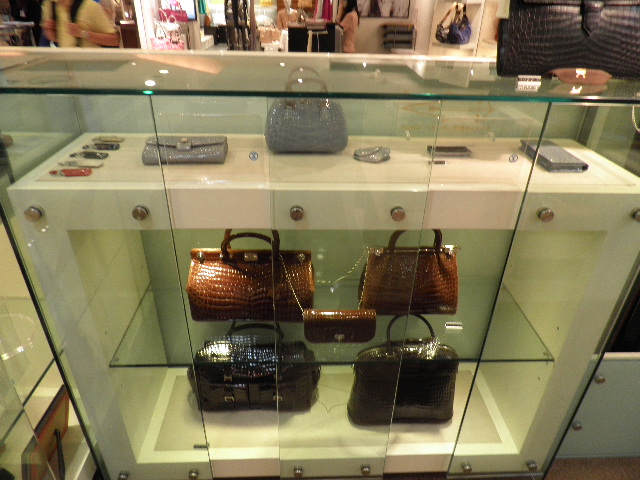This horizontal photograph captures a detailed view inside a boutique, showcasing a prominently lit, glass-encased product display. The display case itself is a white rectangular unit framed by glossy glass panels. Inside, a collection of luxury alligator skin purses is meticulously arranged across three glass shelves.

On the very bottom shelf rest two elegant black purses. The middle shelf features a deep brown ensemble, comprising two purses with a matching brown clutch or wallet positioned in front of them. The top shelf is adorned with a sleek, silver setup: a central purse, accompanied by a matching clutch to its left and a silver wallet to its right.

The display case is illuminated by overhead lights, enhancing the sheen of the purses and highlighting their intricate textures. Additional details include brass-colored knobs on the counter and a brownish glass bowl or plate situated on top.

In the background, the boutique's ambiance is subtly conveyed through the presence of mannequins, additional handbags, and individuals browsing, one notably wearing a pink shirt and another in a green shirt approaching the store. Some small, indistinct items in red, white, black, blue, and possibly silver are also partially visible in the corners of the image.